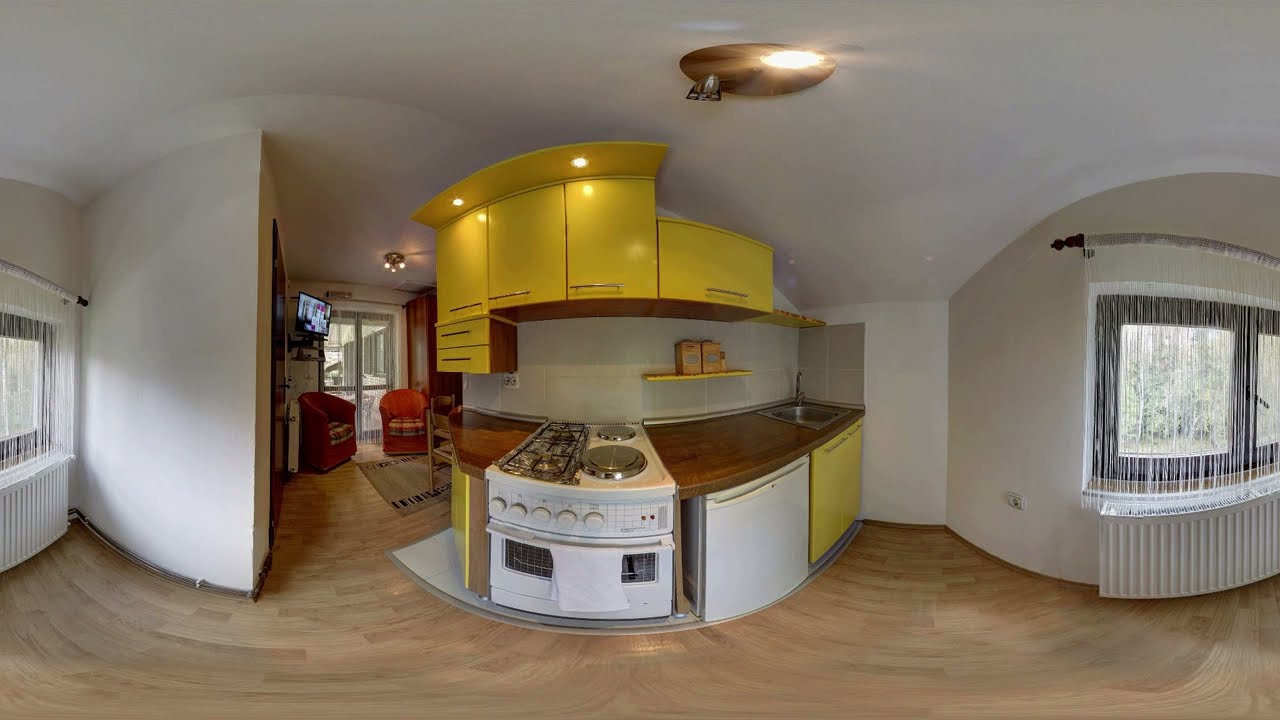This image features a mostly empty studio apartment, captured from the vantage point of the kitchen. The kitchen, which is the focal point of the image, showcases an older theme with distinct yellow cabinets and drawers equipped with chrome U-shaped handles. The countertops are wooden, resembling a cutting board, and there's a small sink situated in the top right corner. A white stove, equipped with a grilled stovetop, two gas burners, and two electric burners, along with a couple of dials, is situated centrally. A white dishwasher is also visible.

The kitchen area is adorned with a shelf underneath the yellow cupboards, holding a few items, likely including some boxes. The apartment has light wooden laminate floors and the walls, along with the ceiling, are painted white. A round copper light fixture hangs at the top of the photo, illuminating the space. 

To the right, there are windows accompanied by a radiator. The background reveals part of the living room area, identifiable by a mounted TV, two flannel-padded red chairs, and a patio window with a tan rug on the floor. The image appears somewhat distorted, giving a panoramic or 360-degree effect, curving some of the lines within the shot.